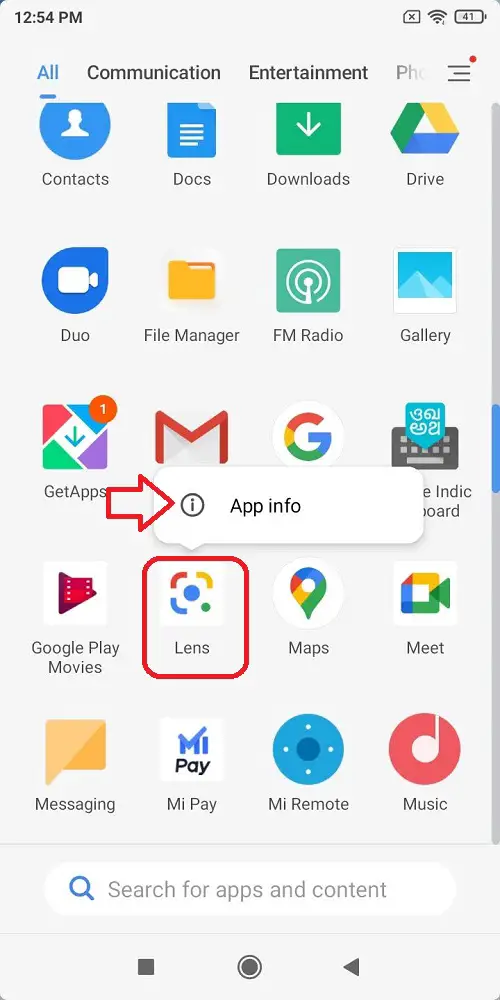**Caption:**

A screenshot of a mobile device interface with a light gray background. At the top of the screen, in bold black text, the time is displayed as 12:54 p.m. To the right of the time, there are icons indicating a notification (a paper with an "X" on it), Wi-Fi signal strength, and battery level at 41%.

Just below the status bar, three tabs are visible: "All" in blue (indicating it's the selected tab), "Communication," and "Entertainment," though the last tab is partially cut off. Additionally, there are three horizontal lines with a red dot to the far right, likely a menu or notification indicator.

The first row of app icons includes "Contacts," "Docs," "Downloads," and "Drive." The second row features "Duo," "File Manager," "FM Radio," and "Gallery." The third row displays "Get Apps," "Gmail," the "Google" app, and a keyboard app that's partially cut off. A white, hollow arrow facing right with an eye inside a circle labeled "App Info" points to the "Lens" app, which is outlined in red, signifying its selection or importance. The remaining icons in this row include "Google Play Movies," "Lens," "Maps," and "Meet."

The bottom row of app icons contains "Messaging," "Mi Pay," "Mi Remote," and "Music." Below the app rows, there is a search box with a blue search icon and the text "Search for apps & content" in light gray.

At the very bottom, the navigation bar has three controls: a solid gray square, two circles (one solid grey and one outlined), and a left-facing triangle, all in gray.